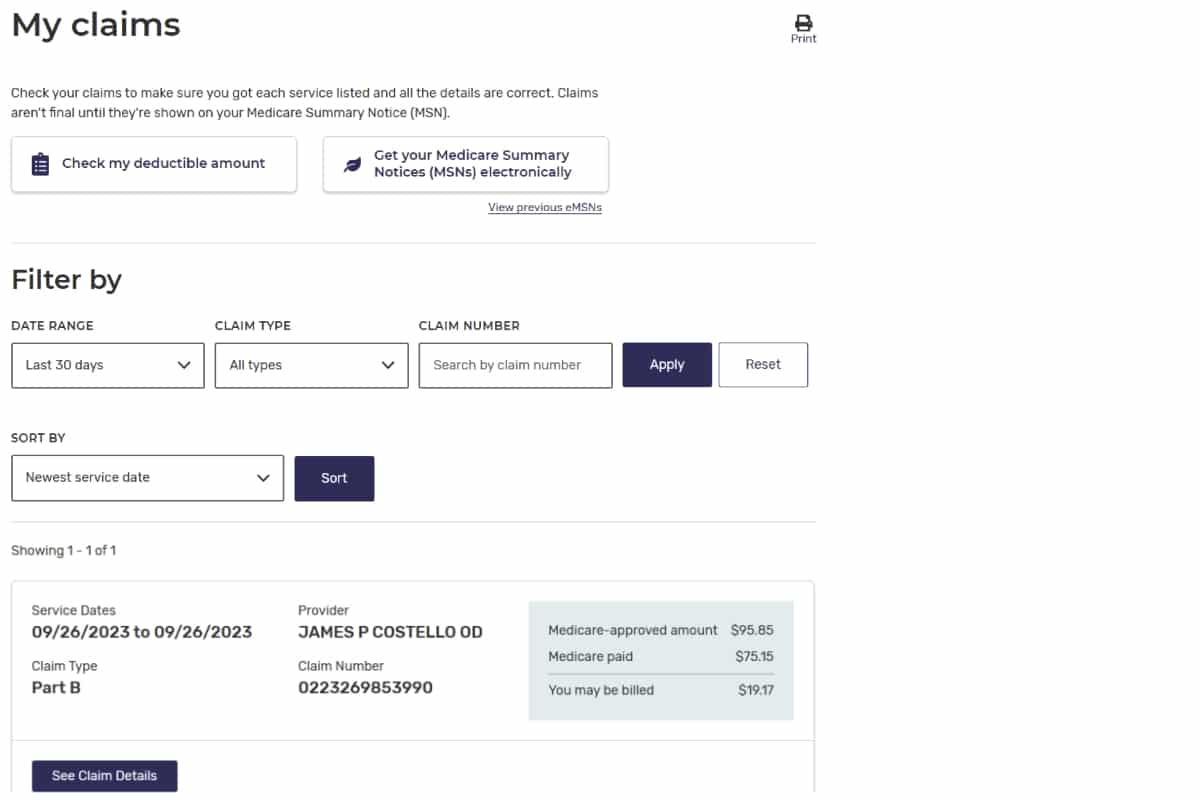This image features a detailed snapshot of a "My Claims" page. At the top, the header reads "My Claims," followed by a description advising users to verify each service listed and ensure all details are correct, as claims are not final until they appear on the Medicare Summary Notice. The page features two prominent buttons: "Check my deductible amount" and "Get your Medicare Summary Notices electronically."

Below this, there is a heading titled "Filter by," which offers various options to filter the displayed claims. Currently, the filters are set to "last 30 days" for date range and "all types" for claim type. There are additional options to search by claim number, with an "Apply" button in blue and a "Reset" button that is clear.

Further down, there's a "Sort By" section, which is currently sorting by the newest service date. A blue "Sort" button is also present. The section below shows "Showing 1, 1 of 1," indicating that there is a single claim listed.

The claim details are as follows:
- **Service Dates:** September 26, 2023, to September 26, 2023
- **Claim Type:** Part B
- **Provider:** James P. Costello, OD
- **Claim Number:** 0223269853990
- **Medicare Approved Amount:** $98,985
- **Medicare Paid:** $75.15
- **You May Be Billed:** $19.17

At the bottom of this section, there is a blue button labeled "See Claim Details."